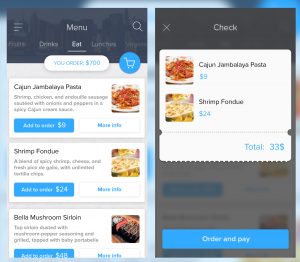The image is a square-shaped frame featuring two side-by-side screenshots from a mobile app. On the left screenshot, menus appear at the top center displaying three identifiable items: "Cajun Jambalaya Pasta," "Shrimp Fondue," and "Bella Mushroom Sirloin." Each menu item has an associated image and an "Add to Order" button beside it, though the smaller text is hard to discern due to the image's reduced size. The right screenshot prominently features the word "Check" at the top. It shows that two items have been selected: "Cajun Jambalaya Pasta" priced at $9, and "Shrimp Fondue" priced at $24. The total amount at the bottom is calculated as $33. The very bottom of this screenshot displays an "Order and Pay" button, which is light blue with white text.